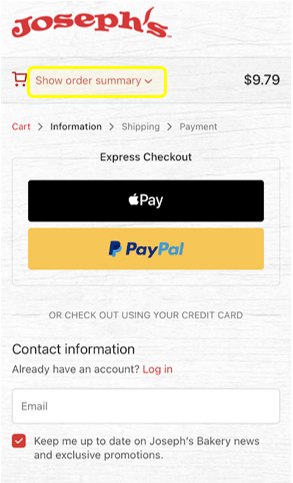The image appears to be a screenshot from a cell phone displaying an online shopping cart summary for "Joseph's." At the top, "Joseph's" is prominently displayed in red text, with a decorative element resembling a red feather in place of a hyphen. Below, a red shopping cart icon accompanies the phrase "Show order summary," also in red, which is enclosed by a yellow rectangle. To the right, the total amount is indicated as $9.79.

Further down, navigation instructions are displayed: "Cart" in red, followed by "Information" in black, "Shipping" in gray, and "Payment" in gray, each with a respective arrow directing towards more details. Below these options is the "Express Checkout" section.

Within the Express Checkout, there are two payment options: Apple Pay and PayPal. Apple Pay features a black background with white text, while PayPal displays a golden-orange background with blue and teal text.

At the bottom of the image, there is a checkbox with the label "Keep me up to date on Joseph's Bakery news and exclusive promotions," highlighted in red, indicating that it is an option for the shopper to subscribe to updates and promotions.